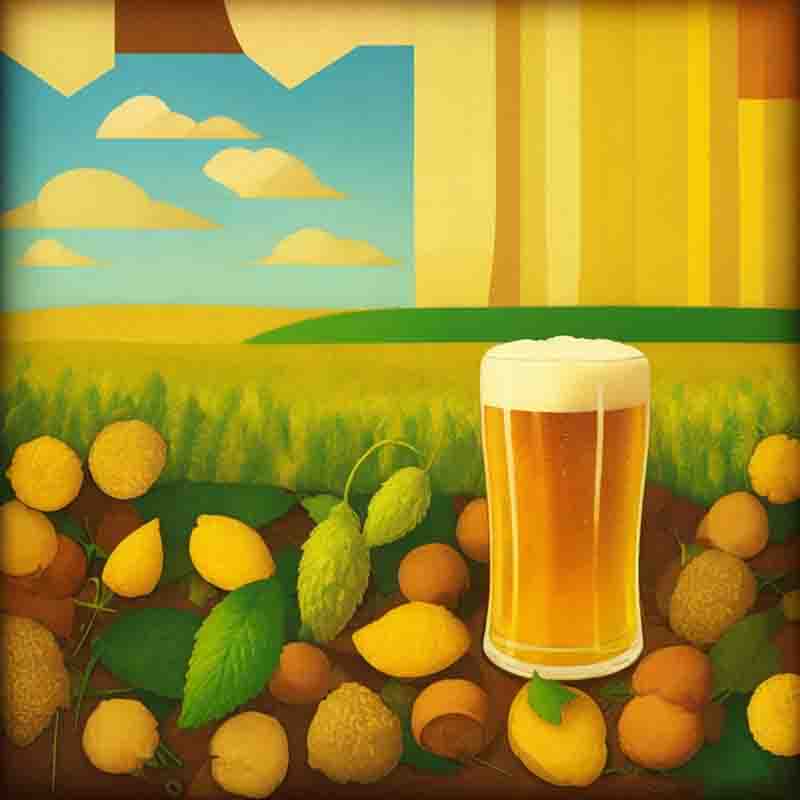The image is a detailed, illustrated painting featuring a serene indoor and outdoor scene. The foreground is dominated by a brown wooden table, adorned with an assortment of fruit, including whole and halved yellow lemons, a tan-colored fruit that could be figs or kiwis, and green leaves scattered among them. To the right side of the table, there is a tall crystal glass filled with a brown liquid topped with white foam, suggesting it might be beer. Near the glass, there's a scattering of more yellow lemons and possibly some small apricots or tangerines.

The room's background includes a window framed with yellow curtains, revealing an outdoor view. Outside, a tranquil landscape unfolds with a blue sky punctuated by white and yellow-tinted clouds. Below, the vibrant green grass, streaked with yellow, is interspersed with tall green and yellow weeds. The window trim is also depicted in brown wood, harmonizing with the table. The overall setting is enriched with a wallpaper featuring yellow and tan stripes, adding to the warm and inviting atmosphere of the scene.